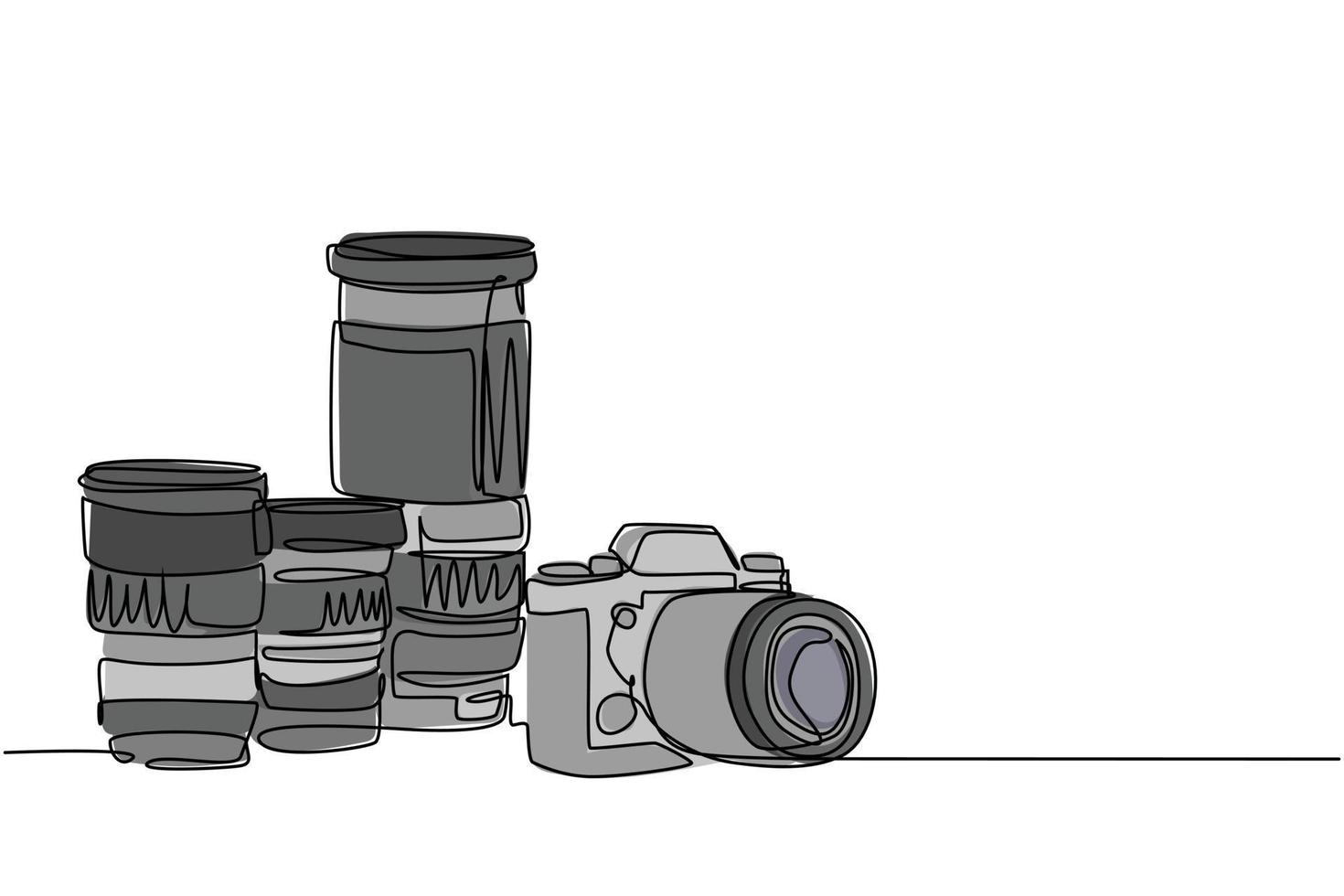This is a detailed black-and-white sketch of a professional-grade SLR (single-lens reflex) camera and its various interchangeable lenses, rendered in a linear, illustrative style with scraggly lines and varying shades of gray. On the right side, the camera body features traditional buttons and controls, with a large cylindrical lens attached, likely a macro lens for close-up shots. To the left of the camera, four lenses are arranged in a row: a large telephoto lens, a medium-sized lens, and another shorter lens, suggesting coverage from telephoto to macro capabilities. The lenses are depicted as cylindrical and dark gray, with one stacked atop two others. This artistic sketch, using a single continuous line, emphasizes the versatility and professional quality of the camera and its accessories.